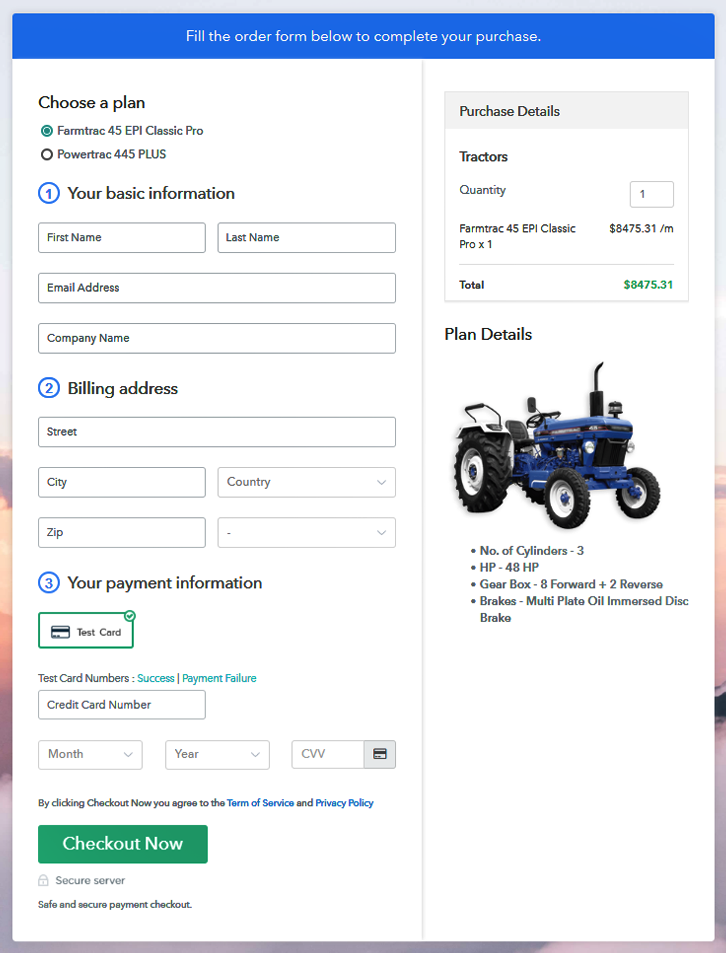**Detailed Checkout Page Description for E-Commerce Tractor Site**

At the top of the checkout page for an e-commerce site specializing in tractors, there's a prominent blue bar containing the instruction: "Fill out the order form below to complete your purchase."

**Plan Selection:**
- **FarmTrack 45 EPI Classic Pro:** This plan is selected by default.
- **Powertrack 445 Plus:** This is another available option but is currently unselected.

**Section 1: Basic Information**
- This section is titled "Your Basic Information," denoted with a blue circle and the number "1" in black text.
- The fields to be filled in include:
  - First Name
  - Last Name
  - Email
  - Company Name

**Section 2: Billing Address**
- Also marked with the number "1" in a blue circle, complementing the previous section.
- Fields include:
  - Street
  - City
  - Country
  - Zip Code
  - An additional blank field, presumably for address line 2 or a special note.

**Section 3: Payment Information**
- A credit card icon labeled "Test Card" appears, with a green rectangle around it, indicating fields for entering card details.
- A note says, "Test card number success and payment failure."
- Payment fields include:
  - Credit Card Number
  - Expiration Month
  - Expiration Year
  - CVV Code
- A green button below states, "Checkout Now – Secure Server," assuring "Safe and Secure Payment Checkout."

**Right Column: Purchase Details**
- Detailed purchase summary:
  - **Tractor:** FarmTrack 45 EPI Classic Pro
  - **Quantity:** 1
  - **Price:** $8,475.31 per month for one tractor
  - **Total:** Displayed prominently in green below the itemized price
- **Plan Details:**
  - A three-quarter shot photograph of the blue tractor accompanies these specifications:
    - Number of Cylinders: 3
    - Horsepower: 48 HP
    - Gearbox: 8 forward and 2 reverse gears
    - Brakes: Multi-plate oil-immersed disc brakes

This organized and detailed layout ensures a user-friendly experience for the customer, guiding them through their purchase process smoothly.